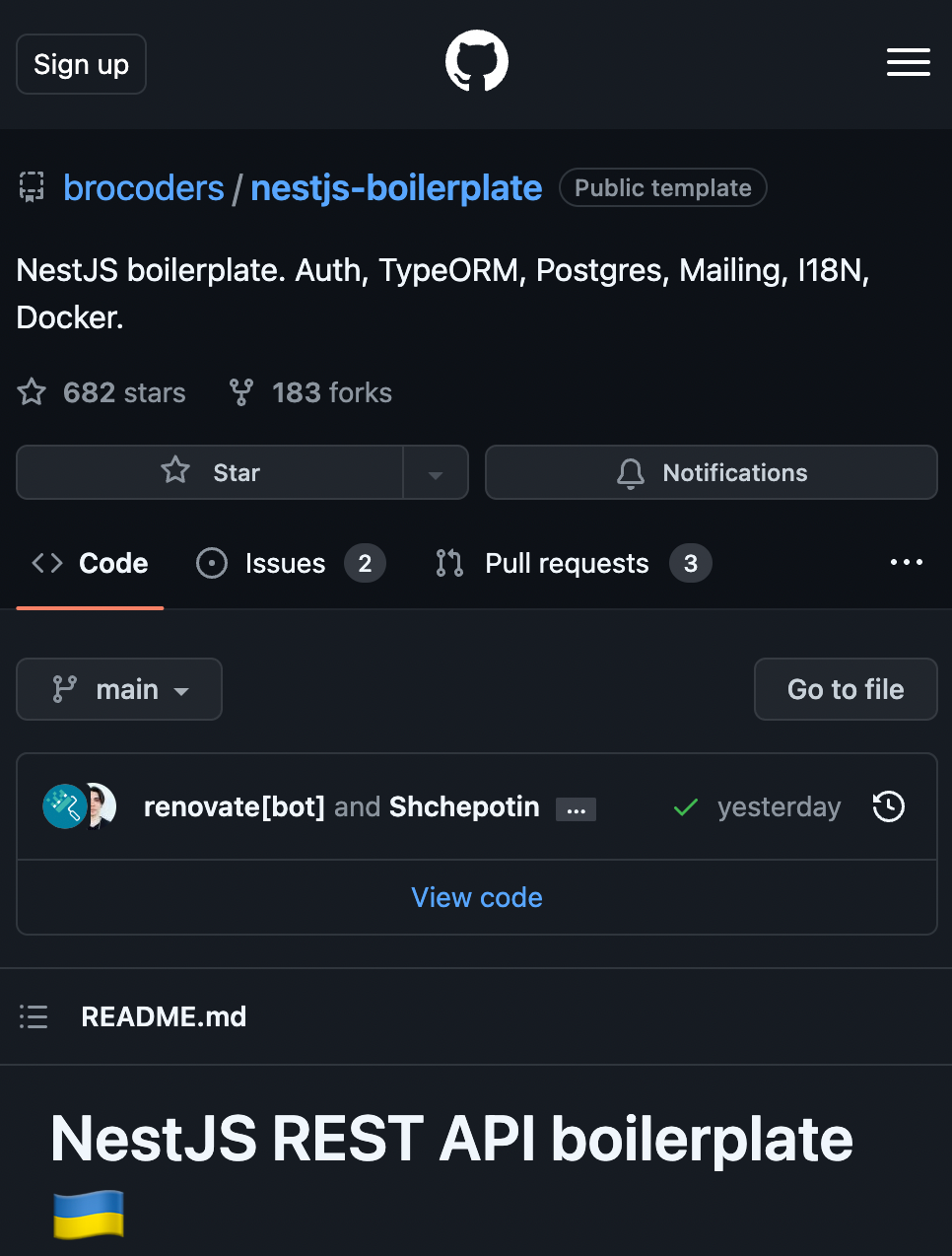The image features a black background, creating a stark and dramatic setting. In the upper left-hand corner, there is a "Sign Up" button, which is also black but is outlined with a thin, bluish light-blue border. The button has squared-off edges and displays the text "Sign Up" in a white font.

At the top center of the image, there is a white circle. Inside this circle is the silhouette of a cat with its left arm extended outward, adding a whimsical touch. Below this circular image, text reads "Brocoders/NestJS-Boilerplate" in white font, providing clarity on the content's source.

To the right of this text, there is a button labeled "Public Template." Beneath this, further descriptive text appears: "NestJS Boilerplate. Auth, TypeORM, PostgreSQL, Mailing, i18n, Docker." This list of technologies and features highlights the robust capabilities of the template.

At the very bottom of the image, a final line of text states "NestJS REST API Boilerplate," underscoring the purpose and functionality of the template.